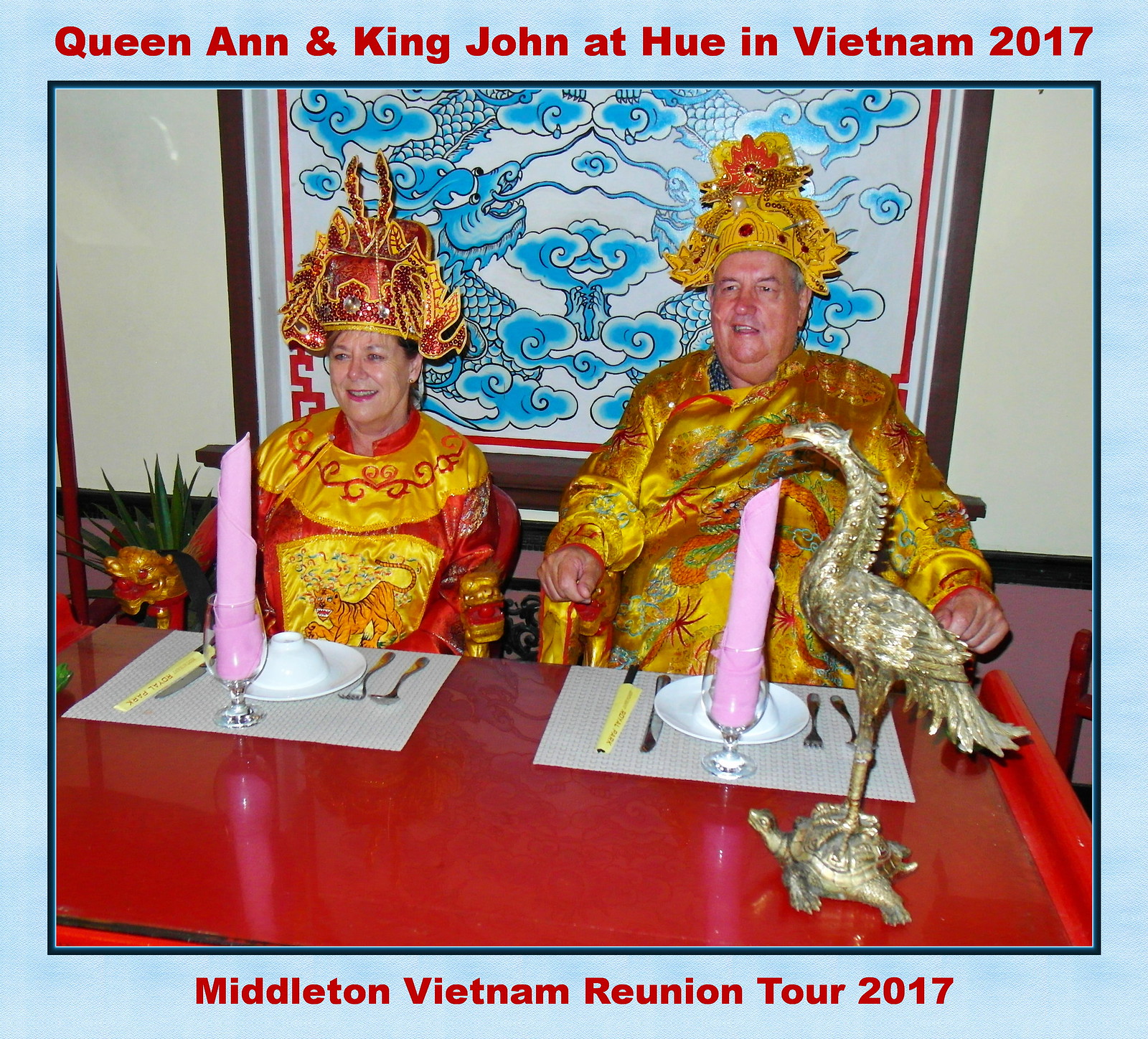This photo captures a man and a woman, both Caucasian, dressed in elaborate ceremonial Japanese attire. They are seated at a very ornate red table, adorned with a bronze sculpture of an animal, either a dragon or a peacock, perched on a turtle. In front of them, the table is set with placemats, utensils, plates, and glasses, each with a pink napkin elegantly arranged inside. 

The woman, seated on the left, is wearing a splendid gold robe with red highlights, featuring a detailed tiger embroidery on her chest. Her attire includes a gold collar and red crown embellished with decorative beads, sequins, and jewels. The man, seated on the right, dons an equally impressive gold robe adorned with dragon designs and complemented by a gold crown decorated with beads.

Behind them hangs a striking tapestry in blue and white, depicting dragons among clouds. This tapestry adds a majestic backdrop to the image. The photo is framed with a blue banner that reads in red letters at the top, "Queen Anne and King John at Hieu in Vietnam 2017," and at the bottom, "Middleton Vietnam Reunion Tour 2017."